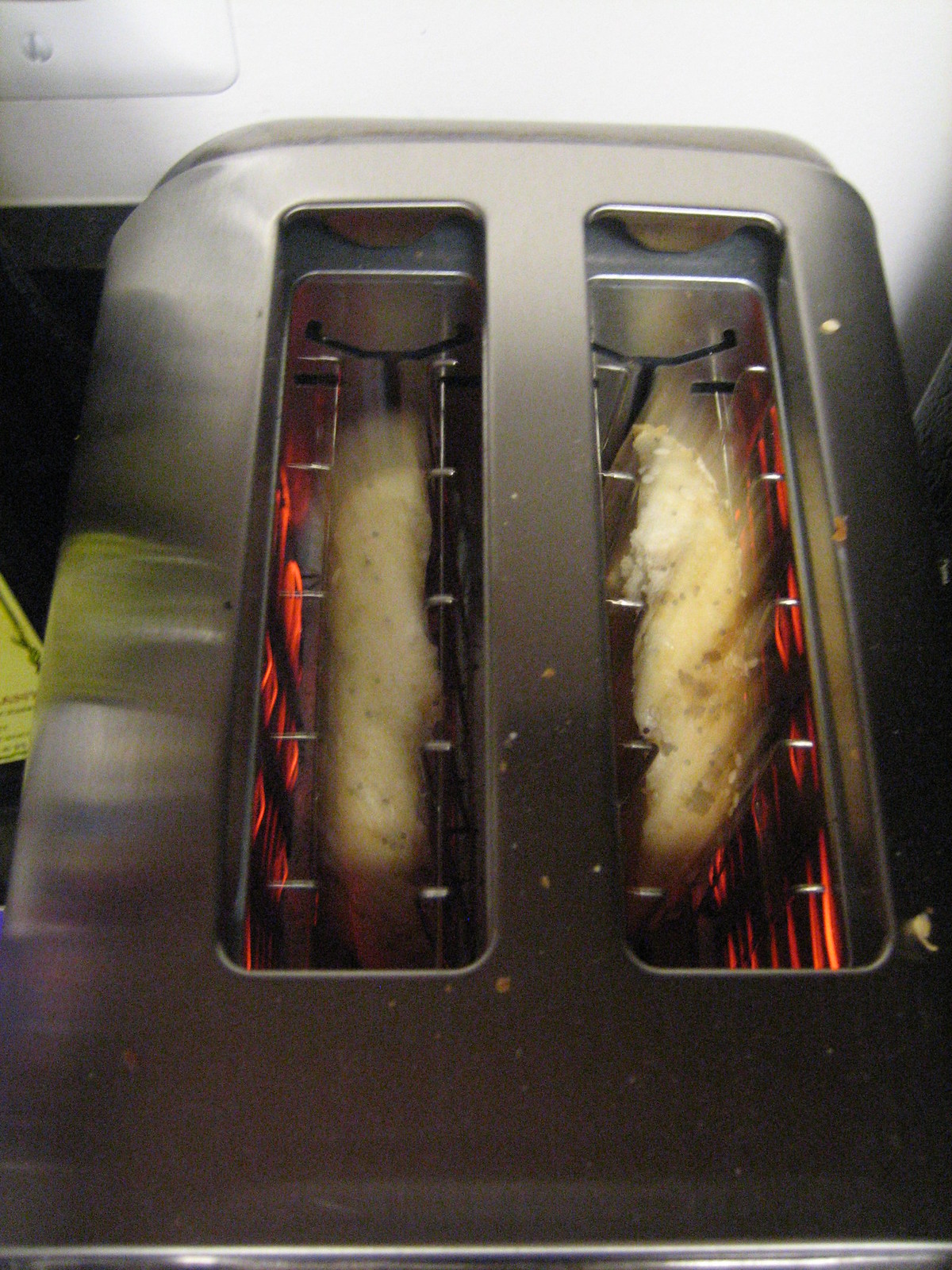This is a detailed, close-up photo of a stainless steel toaster viewed from above, prominently positioned against a mixed background with a white wall and a portion of a black backdrop with a partially visible yellow label. The toaster, which can hold up to two slices of bread, currently contains a bagel, possibly an everything bagel as indicated by the visible sesame seeds and green flakes. The heating coils inside the toaster are glowing red-hot, actively toasting the bagel that appears to have just begun the toasting process, based on its pale color. The surface of the toaster is scattered with crumbs from previous uses. The electrical outlet behind the toaster is just visible, along with part of the backsplash, but the dominant focus remains on the toaster and its contents. The image suggests a sense of motion with a slight blur, as if the bagel was in the middle of being lowered when the photo was taken.